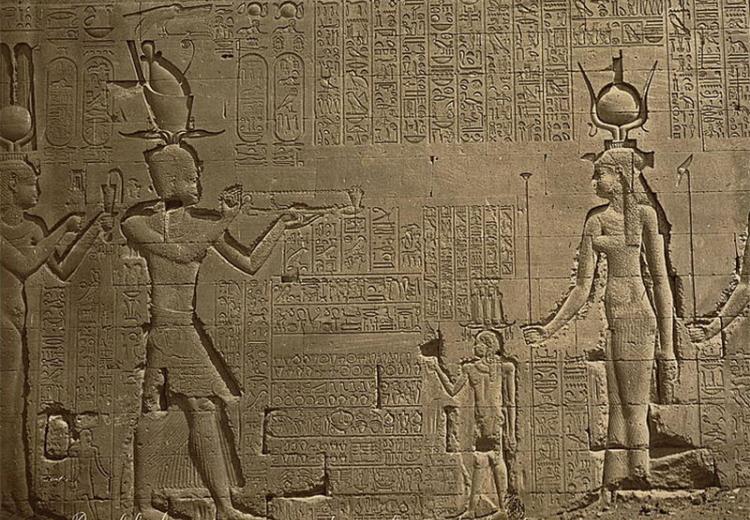The image depicts an intricate scene from ancient Egyptian art, featuring a series of figures adorned in traditional attire and accessories. On the left side of the image, there are two men, both walking to the right. The first man, partially cut off at the left edge of the illustration, holds a whip-like object in his hand and dons an elaborate hat crowned with a spherical ornament. The second man, situated to the right of the first, is wearing a large, corn-shaped headdress. He holds a cup in one hand and a dish containing an unknown substance in the other.

To the right of these men stands a child facing them, wearing a hat adorned with candle-like shapes and holding a black hat. Further to the right is a woman who gazes towards the left. She gestures with an open palm using her left hand while her right hand rests by her side. She, too, is wearing a distinctive headdress and has both hands supporting a large spherical object. The very edge of the illustration shows an enigmatic hand extending from the right towards the center of the scene, adding to the mystique of the composition. Hieroglyphic text accompanies the drawing, providing context or narrative to the represented figures.